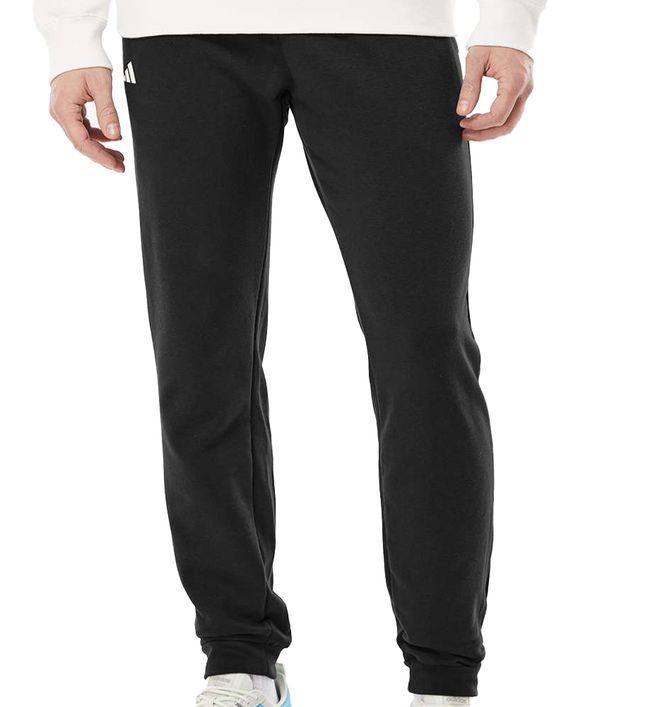The image depicts a person standing against a white background, captured from just above the waist down to the feet. The individual is wearing a white long-sleeved sweater and dark-colored sweatpants, which appear loose but gather tightly around the ankles. The person's hands are relaxed at their sides, with slightly curled fingers, and the thumbs facing forward. The sweatpants feature a noticeable logo on the right hip, identified as the Adidas symbol. The person's legs are relatively thin, and the weight appears to be predominantly on the right foot, as the left knee is slightly bent. The footwear consists of white sneakers with a small blue detail on the left shoe, while just the edge of the right shoe is visible.